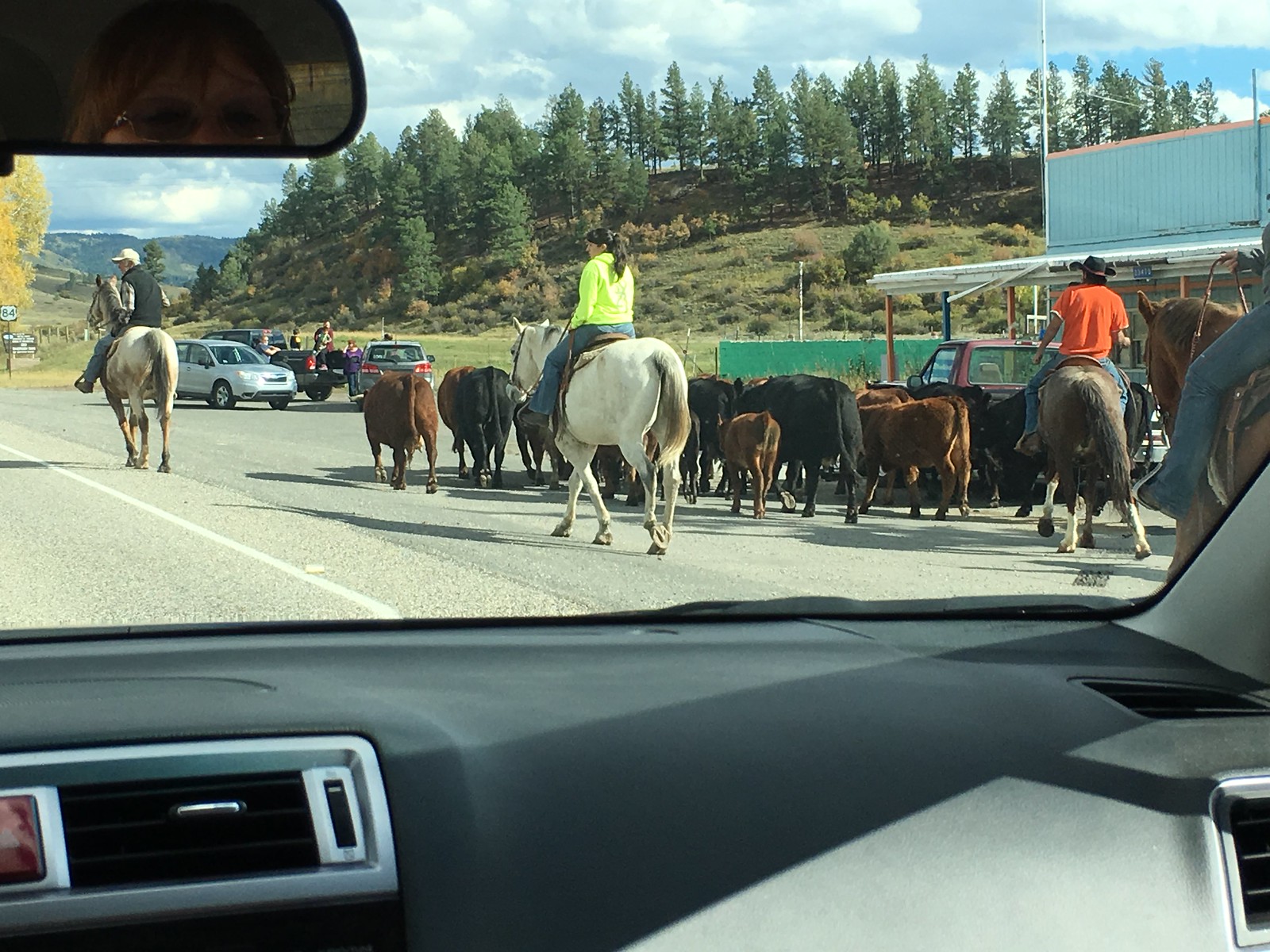A vibrant scene captured from inside a vehicle through a front windshield reveals a picturesque countryside. The interior of the vehicle is showcased with a gray dashboard in the foreground. Beyond the windshield, a sprawling blue sky stretches across the background, crowned by a scenic hill adorned with lush green grass and a dense array of evergreen trees. The highway, which appears to be gray in color, unfolds ahead, providing a unique setting where three horse riders, and possibly a fourth partially cut-off rider, are herding a group of cattle along the road.

On the left, a man rides a white and tan horse, fully visible and poised in action. At the center, a woman with dark hair tied in a ponytail and wearing a chartreuse hoodie paired with blue jeans rides atop a majestic white horse with a gray mane and tail. On the right, a man dressed in an orange shirt rides a sturdy brown horse adorned with distinctive white feet.

The cattle, moving forward and only showing their rumps in the photograph, include a mix of small and large animals, exhibiting different hues of dark brown and black coats. A few more vehicles are visible in the distance, adding a modern contrast to this pastoral scene on the blacktop road.